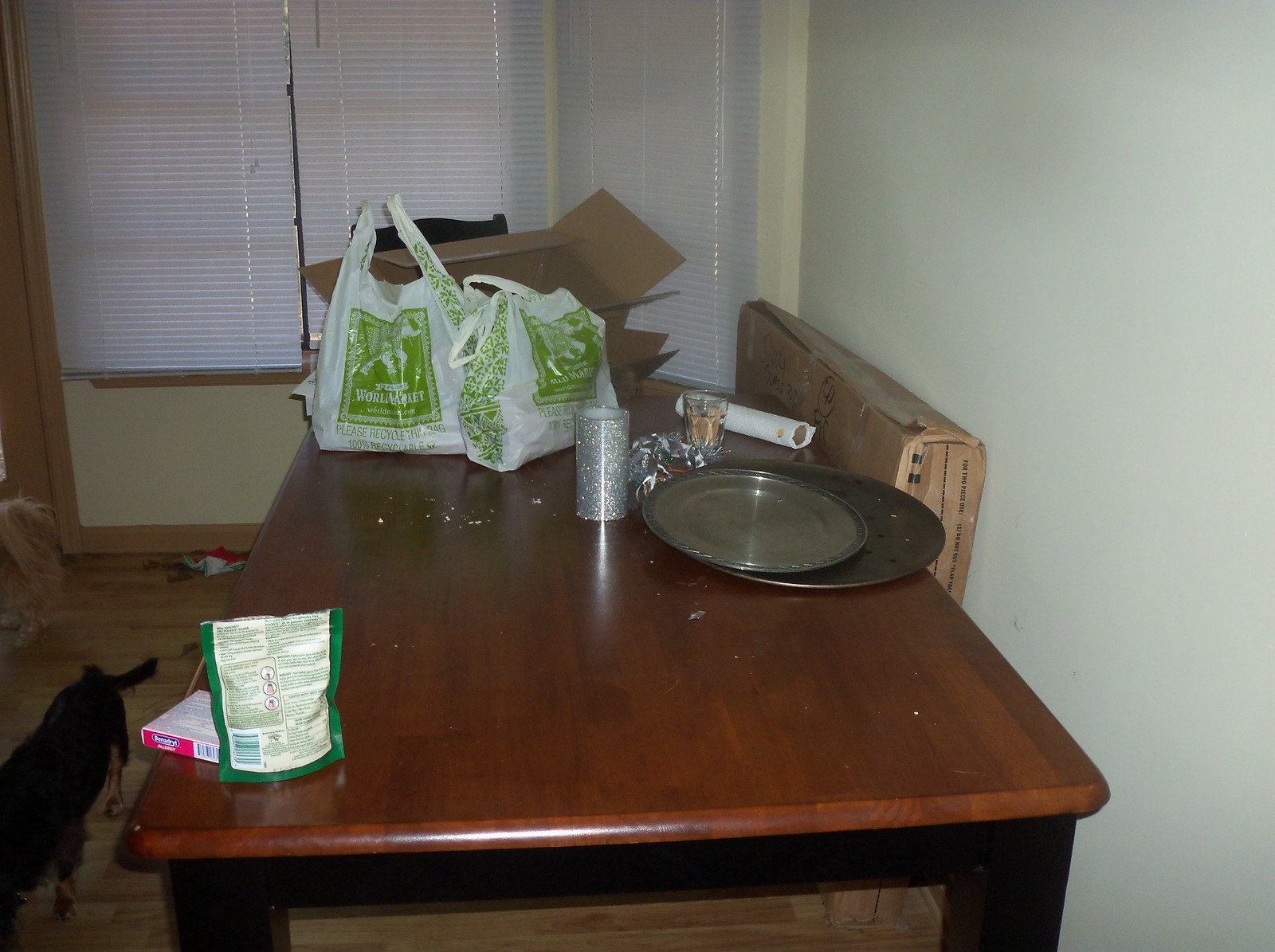In this dimly lit photograph, a wood-topped table with black, likely wooden, legs stands approximately 8 inches from a light green wall on the right. Against this wall leans a large cardboard box. In the background, a slightly elevated window is adorned with at least three mini blinds, partially revealing more of the green wall to the left of the table. On the floor, there is a small black and brown dog, though only its feet and tail are visible. The floor appears to be pine wood, adding a rustic touch to the setting. 

The surface of the table is cluttered with various items: a couple of round metal plates, several white and green plastic bags, a small box, a pouch that seems to contain dog treats, and a stack of cardboard. The overall atmosphere is somewhat shadowy, making detailed observation challenging.